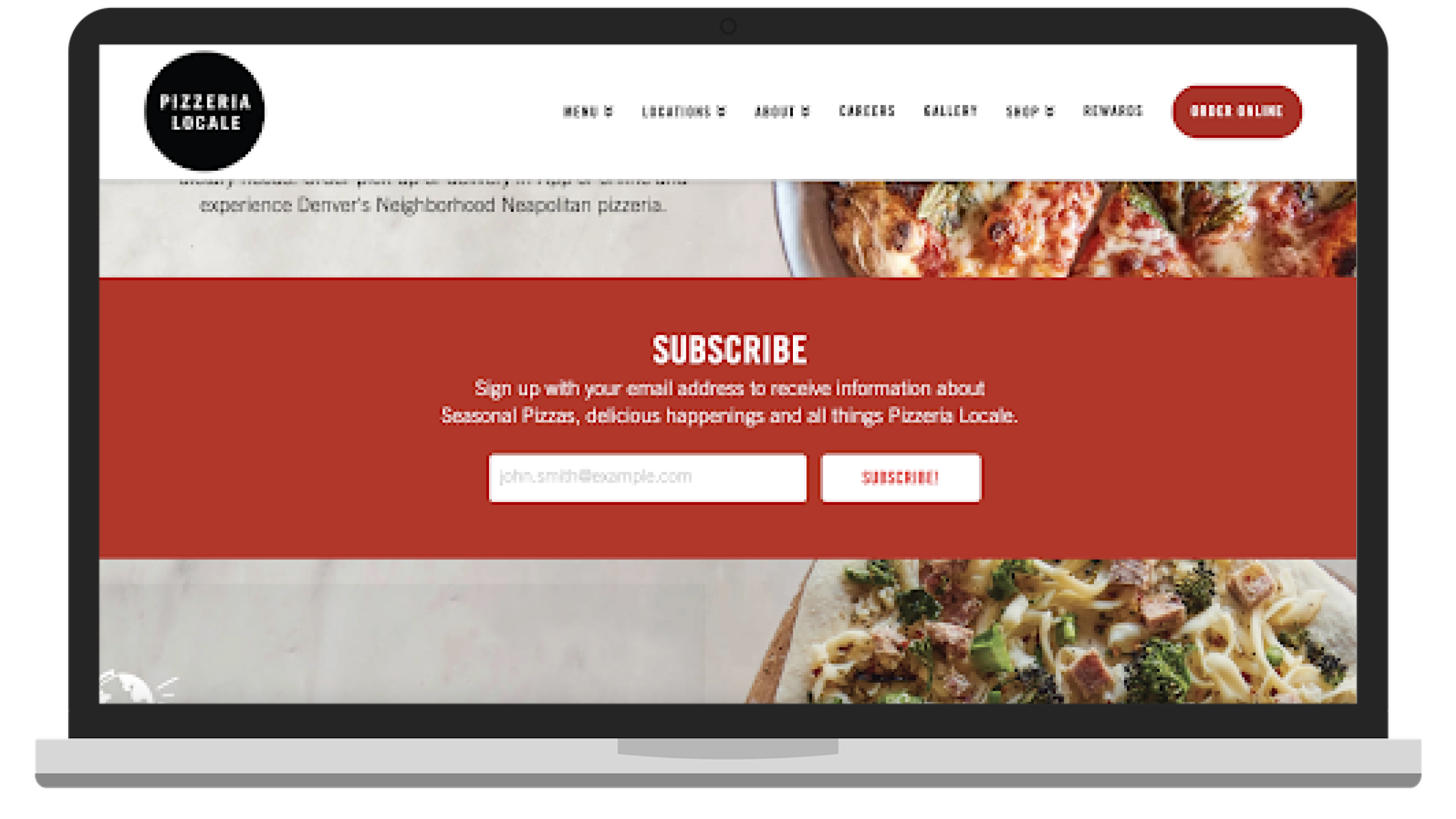This image is a screenshot of what appears to be the homepage of a website. At the very top, the navigational menu is set against a clean white background. In the upper left corner, a black circle encloses the text "Pizzeria Locale" written in white. Moving from the center towards the right side of the menu, the navigational items listed are: Menu, Locations, About, Careers, Gallery, Shop, and Rewards. On the far right, an eye-catching red oblong button with rounded corners features the text "Order Online" in white.

Dominating the main section of the webpage is a large rectangular banner in a brick-red hue. This banner contains a subscription prompt in white text, stating: "Subscribe. Sign up with your email address to receive information about seasonal pizzas, delicious happenings, and all things Pizzeria Locale." Below this text, there is a white rectangle for users to input their email address, adjacent to another white rectangle with the text "Subscribe."

This red subscription banner partially overlays a food photograph. At the top of the image, a tantalizing pizza is visible, showcasing its appealing toppings. At the bottom, there is a pasta dish featuring noodles, beef, and broccoli, suggesting a hearty and flavorful meal.